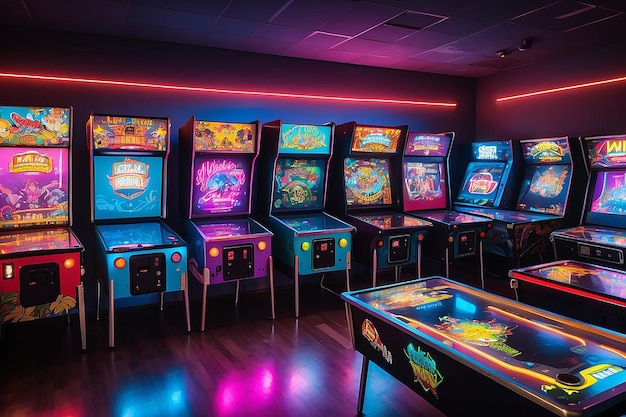The image depicts a hyper-realistic arcade room illuminated by a vibrant array of neon colors. Lined up against the walls are twelve diverse pinball machines, each glowing in hues of neon pink, blue, and green. A thin, continuous neon line stretches across the top of the wall from the left corner to the right, adding to the room's vibrant atmosphere. The arcade features a highly reflective wooden floor that mirrors the colorful lights from the machines. In the middle of the room, there is an ice hockey table. The primary colors in the image include dark orange, teal blue, dark mauve, dark red, white, navy blue, and dark yellow, enhancing the vivid and lively ambiance of this classic game parlor.